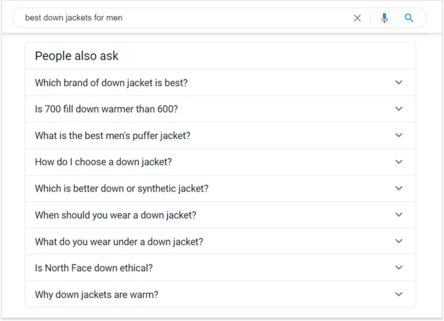This image is a detailed screenshot of a search results page from an online query about the "best down jackets for men." At the very top left corner within the search bar, the query "best down jackets for men" is visible. On the top right corner, there are two icons: a magnifying glass for search and a microphone button for voice search. Immediately below the search bar, the heading "People also ask" is prominently displayed in black letters.

A vertical list on the left side of the screen shows related queries people frequently ask:
1. Which brand of down jacket is best?
2. Is 700 fill down warmer than 600?
3. What is the best men's puffer jacket?
4. How do I choose a down jacket?
5. Which is better, down or synthetic jacket?
6. When should you wear a down jacket?
7. What do you wear under a down jacket?
8. Is North Face down ethical?
9. Why are down jackets warm?

Each of these questions has a clickable drop-down arrow on their right side, presumably to reveal further details or answers. The screenshot captures the search interface cleanly and clearly, outlining the main options and related popular queries users might explore.